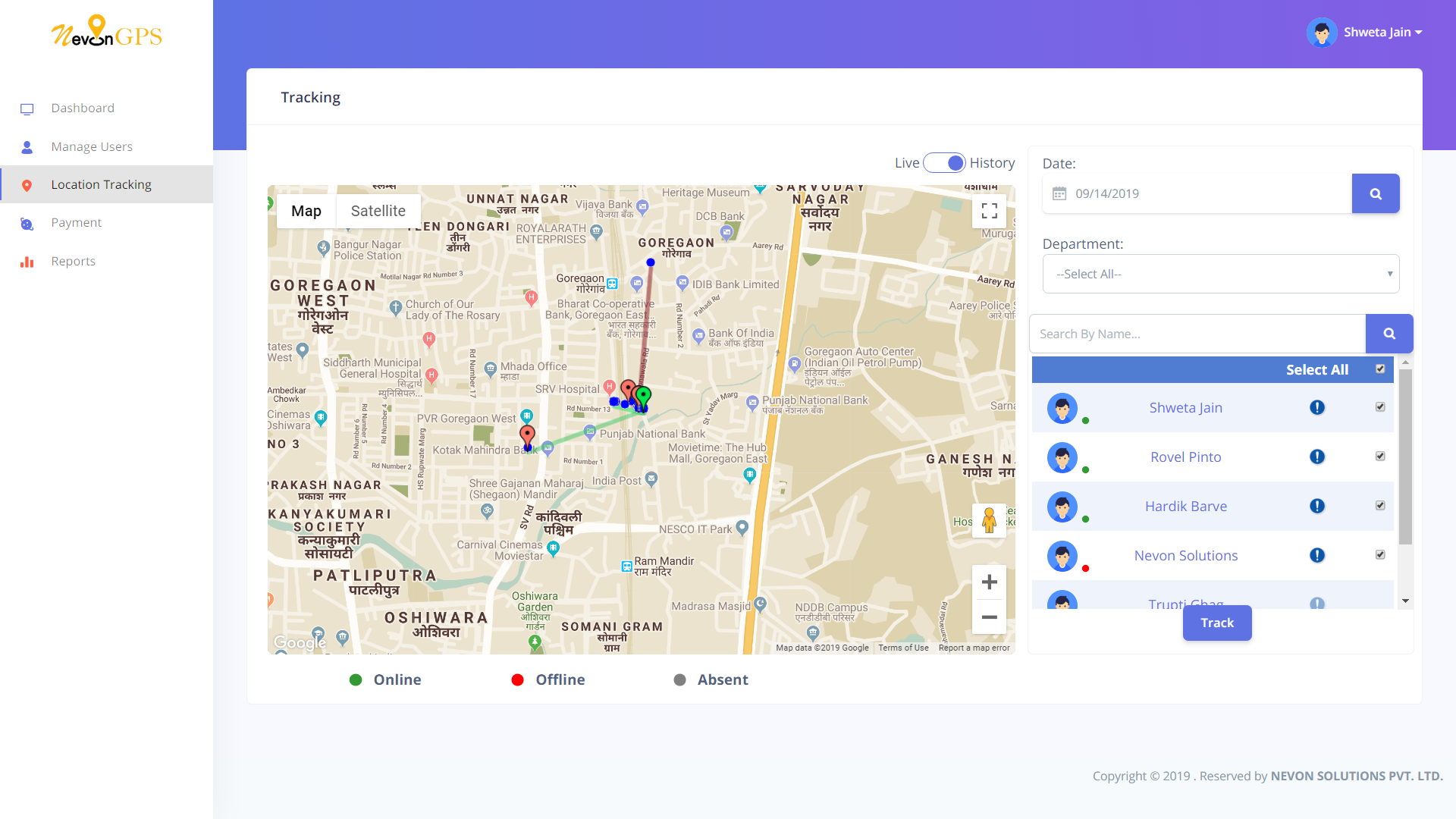The image is a screenshot of a website, presented in a zoomed-out view, making most of the text difficult to read. The main body of the site has a white background. The top segment of the site features a gradient background, transitioning from lilac on the left to purple on the right, with a pale gray section below. 

In the top left corner, above the left navigation panel, there is a yellow logo featuring a map pin icon accompanied by text that is largely unreadable, although it appears to include "GPS". On the top right corner, within the purple section of the banner, there is a profile picture in a circular frame alongside a name and a drop-down menu.

Below the logo, there are five navigation options, but the text is too small to distinguish. The main screen of the website displays a header that reads "Tracking" above a map. This map shows roads, various pins, and what seems to be a travel route. A key indicates the status of vehicles with green dots for online, red dots for offline, and gray dots for absent. This suggests the platform is used for tracking company vehicles.

The map includes locations such as Oshiwara and Patliputra, hinting that the site may pertain to a region in India. On the right side, adjacent to the map, there are options for selecting the date, department, and a search bar. Below these options, a section lists different drivers along with their names and status indicators (online, offline, or absent), each accompanied by a "track" button.

In the bottom right corner, there is some copyright information attributed to "Nevon Solutions Pty Ltd."